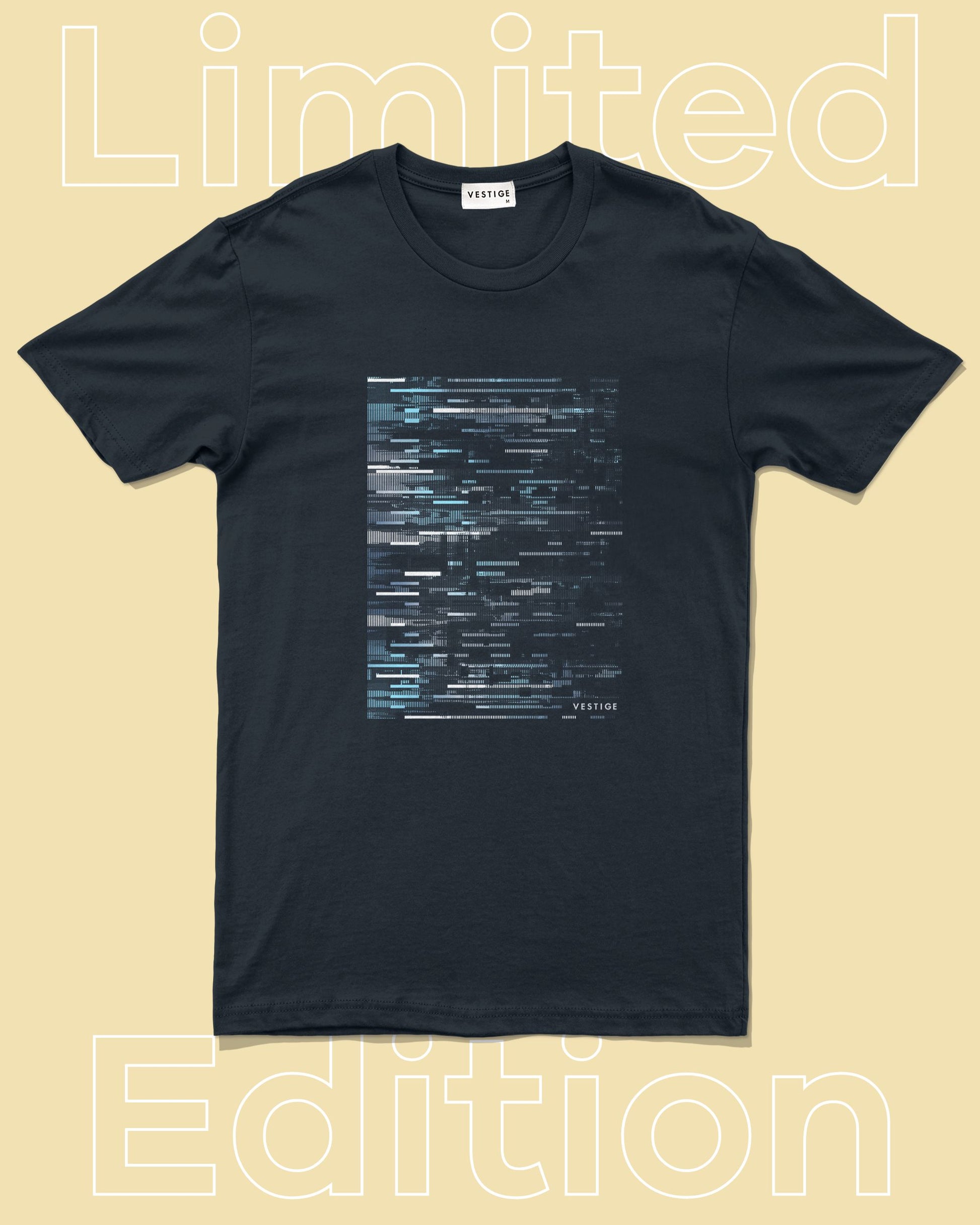This is a rectangular image that is taller than it is wide, with a beige or cream-colored background. Displayed in outlined white block letters at the top and bottom of the image, it reads "Limited" and "Edition," respectively. The main focus of the image is a black, short-sleeved cotton t-shirt. Inside the collar, there is a white label that reads "Vestige" in black text. The front of the t-shirt features an abstract design in a rectangle shape, also taller than it is wide, consisting of variegated lines in shades of blue, white, and black. This design resembles static or a glitching computer screen. In the bottom right corner of the design, "Vestige" is printed in white text.